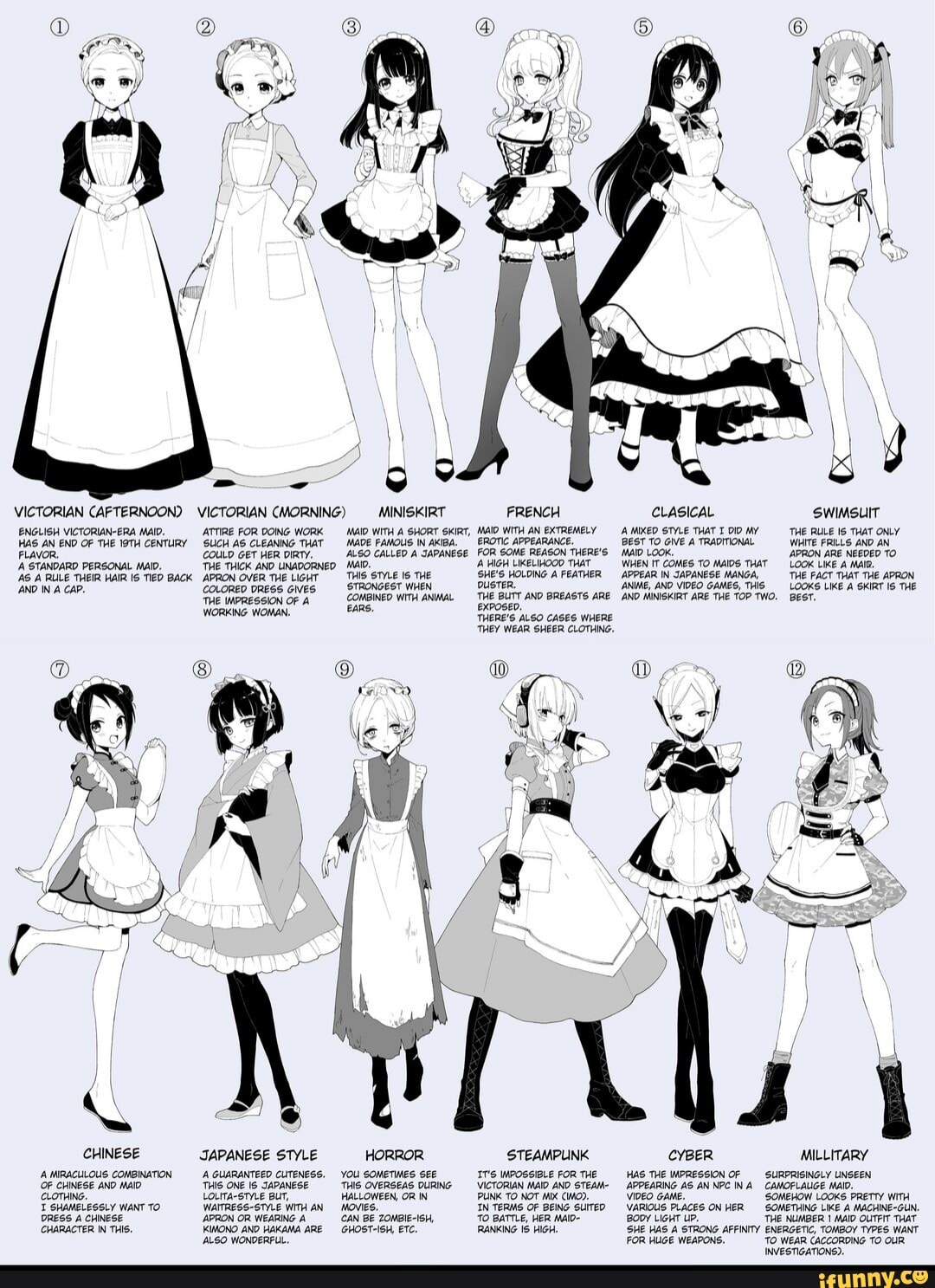The image is a detailed catalog-like illustration showcasing 12 distinct anime characters, each donning a unique maid uniform or costume. These grayscale drawings are arranged in two rows of six characters, set against a light bluish-gray background. Each character is labeled with the name and description of her outfit, such as Victorian (Afternoon), Victorian (Morning), Miniskirt, French, Classical Dress, Swimsuit, Chinese Dress, Japanese Style, Horror, Steampunk, Cyber, and Military. The characters are depicted with various hairstyles and accessories, ranging from long and short to curly, pigtailed, and loose styles, reflecting each character's unique personality. At the bottom, the image is branded with "iFunny.co" in yellow, featuring a smiley face symbol in place of the 'O'. The detailed grayscale shades of white, black, and gray enhance the visual appeal, emphasizing the distinct features of each costume and character.